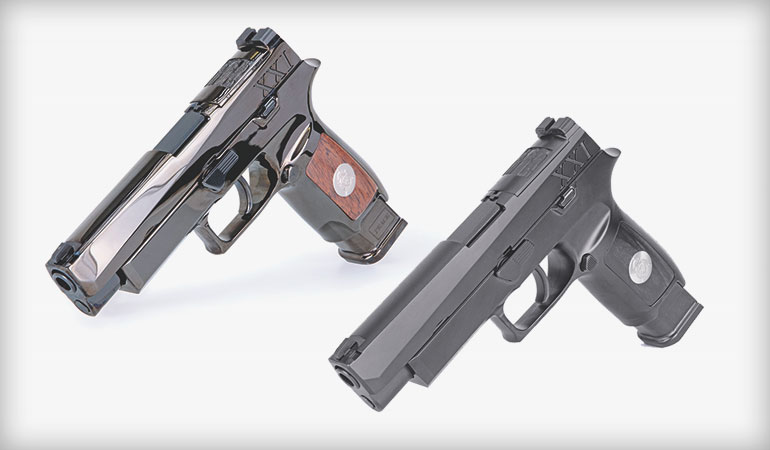The image shows two handguns arranged side-by-side in a horizontal rectangular frame against a light gray background. Both guns are dark gray steel, with the handles oriented towards the upper right corner and the barrels towards the bottom left. The gun in the foreground features a polished wooden handle with a light gray circular emblem embedded in the center. The other gun has a more consistent dark gray finish, including a black area where the wood would be, also adorned with a similar light gray circular emblem. Both firearms display the Roman numeral XXI on their top side and include visible safety mechanisms next to the triggers. The positioning of the guns forms an inverted V shape, with both handles and nozzles touching the surface.